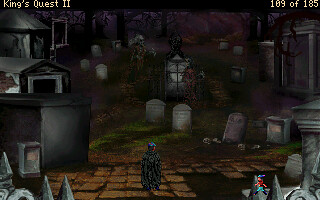In this captivating still from the classic 8-bit video game "King's Quest 2," the scene is set in a graveyard shrouded in the darkness of night. The top of the screen features a narrow black bar displaying white text that reads "King's Quest 2" on the upper left and "109 of 185" on the upper right. 

Dominating the center of the image is a fearsome knight clad in black armor, distinguished by an aqua-tinted helmet adorned with striking red accents. He wields a formidable blade, poised for battle amidst the eerie graveyard's gray stone crypts, tombs, and gravestones.

In stark contrast, towards the lower right corner, stands a diminutive figure about one-third the size of the knight. This small character dons an aqua hat with a feather, a red shirt, aqua pants, and black shoes, adding a touch of vibrant color to the somber surroundings. The detailed pixel art evokes nostalgia, highlighting the intricate design and atmospheric setting typical of early video gaming.